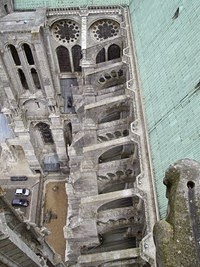This image appears to be a full-color digital rendering, evocative of a computer animation or video game style, providing a bird's-eye view of a Gothic cathedral that resembles the iconic Notre Dame in France. Captured from above, the focus is on the cathedral's light green, sloped roof situated towards the right side of the image, adorned with teal tiles and intricate gray stone gutters or edging. Alongside the roof, we see gray stone buttresses and potentially a small gargoyle figure, enhancing the Gothic architecture's authenticity. On the left side of the image, below the cathedral, there is a brown brick or stone walkway where two cars are parked adjacent to the structure; one car is white or silver, and the other is a dark blue or black color. The composition emphasizes the detailed and textured elements of the cathedral's roof and surrounding architecture, juxtaposed with the mundane scene of parked vehicles below.